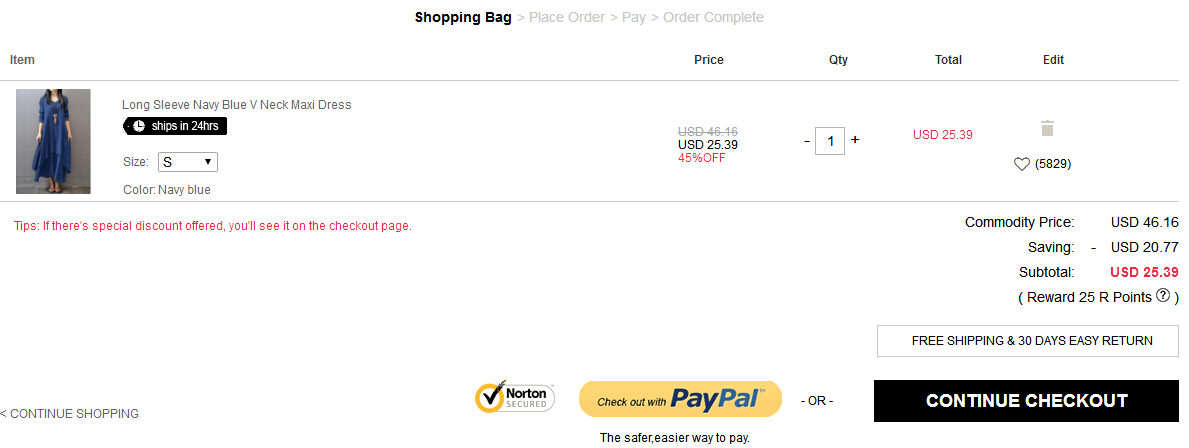**Detailed Caption:**

The image depicts a checkout screen from a shopping app with a clean, white background in landscape orientation. At the top of the screen, a breadcrumb navigation trail is visible, showing the following sequence: "Shopping Bag" followed by a right arrow, "Place Order" followed by a right arrow, "Pay" followed by a right arrow, and "Order Complete." The current page displayed is the "Shopping Bag" section.

Below the breadcrumbs, there is a table with headers labeled as follows from left to right: "Item," "Price," "Quantity," "Total," and "Edit." 

In the first row under the "Item" column, there is an image of a woman wearing a long sleeve, navy blue V-neck maxi dress. The description states the dress will ship within 24 hours and mentions the selected size is S (small), with the color being navy blue.

Under the "Price" column, the original price listed is crossed out, showing "USD 46.16." Beneath the crossed-out price, a sale price "USD 25.39" is highlighted in red, indicating a 45% discount.

In the "Quantity" column, a box is flanked by plus and minus symbols, with the current quantity set to "1."

The "Total" column shows the total cost of the item in red, "USD 25.39."

In the "Edit" column, there’s a trash can icon presumably for deleting the item from the cart, and a small heart icon with the number "58.29" in parentheses next to it, possibly indicating the item's popularity or rating.

Below the table, to the left, there is a note stating: "Tips: If there’s a special discount offered, you’ll see it on the checkout page."